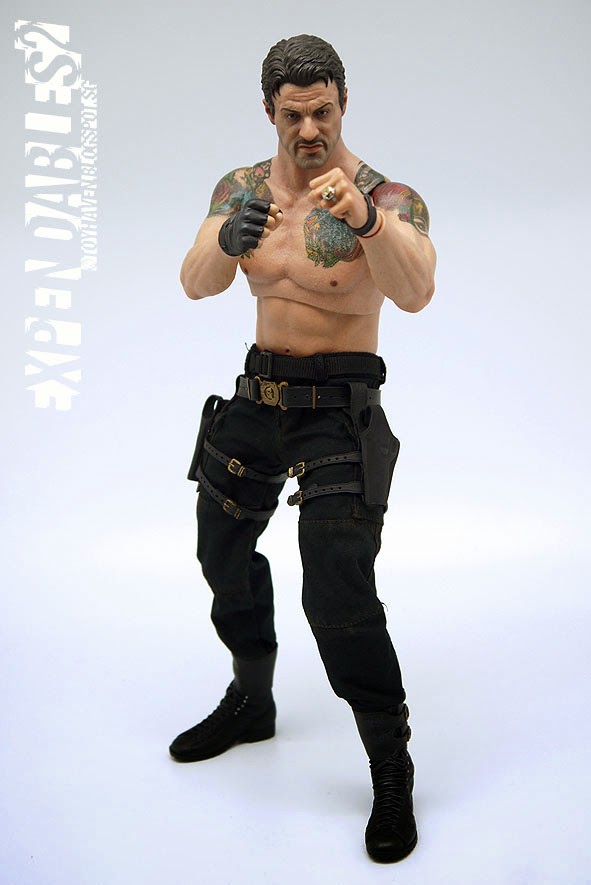The image showcases a detailed action figure of Sylvester Stallone, iconic for his role in "The Expendables." The muscular figurine, depicted with an aggressive, fight-ready pose, features clenched fists and an intense facial expression. His attire consists of black cargo pants adorned with leather buckles and straps, black boots, and gun holsters strapped to each leg. The Stallone figure is shirtless, revealing colorful green and red tattoos on both his upper biceps, shoulders, and the left side of his chest. He sports a black fingerless glove on his right hand and a black bracelet or strap on his left wrist, which also has a ring on the ring finger. The word "Expendables" is visible on the left side of the image, set against a bluish-gray background, suggesting a promotional or advertisement setting for the action figurine.